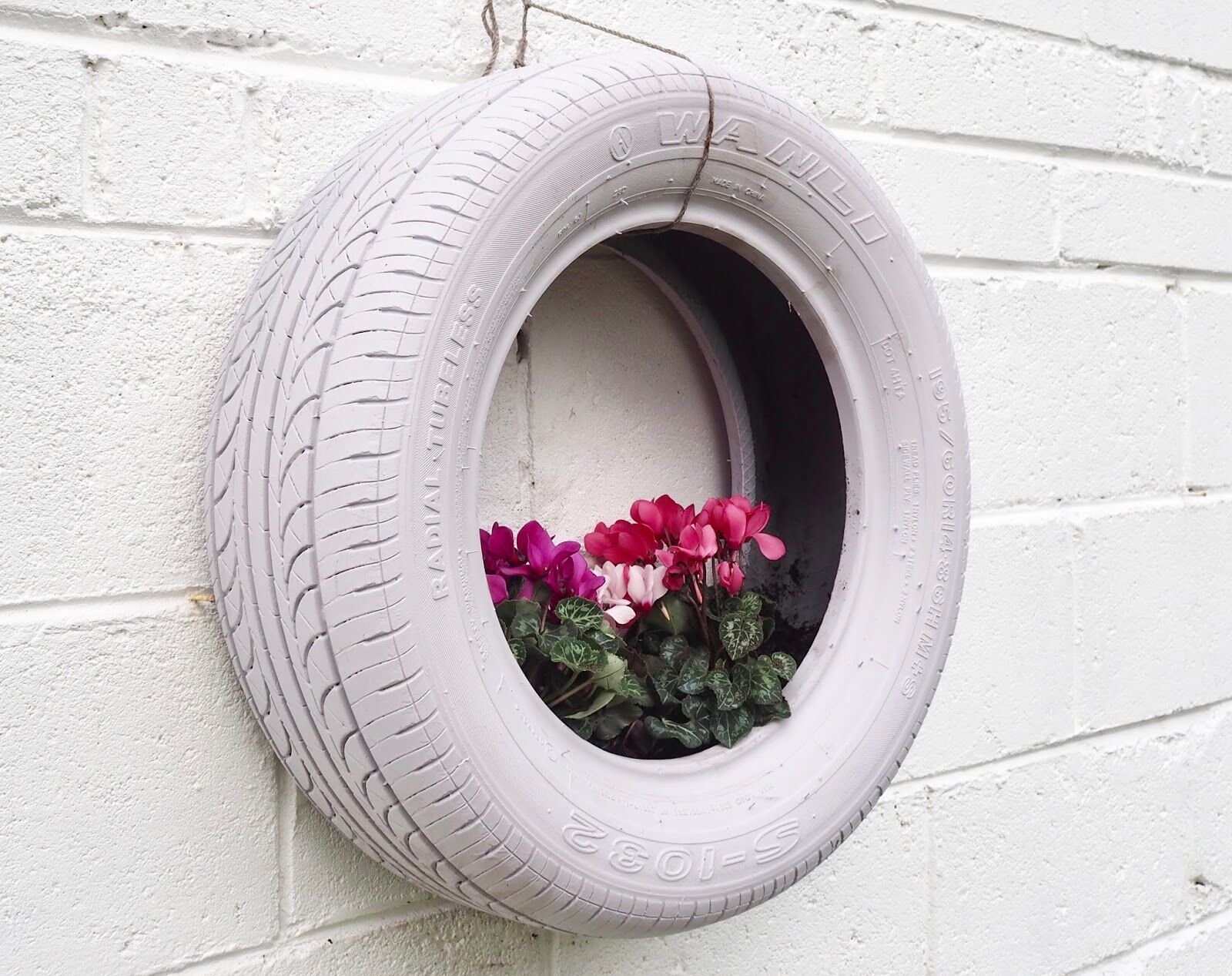This photograph captures a creatively repurposed tire, painted white and suspended on a white cinder block wall using beige twine. The tire, originally intended for a car, has been defunctionalized and transformed into a decorative planter. The brand name "WANLI" and the text "radial tubeless S-1032" are imprinted on its side, hinting at its former life. Nestled within the tire are vibrant flowers of varying shades—pink, lavender, and reddish hues—complemented by green leaves with lighter green centers. The entire scene is a striking juxtaposition of utilitarian and aesthetic elements, showcasing how ordinary objects can be repurposed into charming decor.